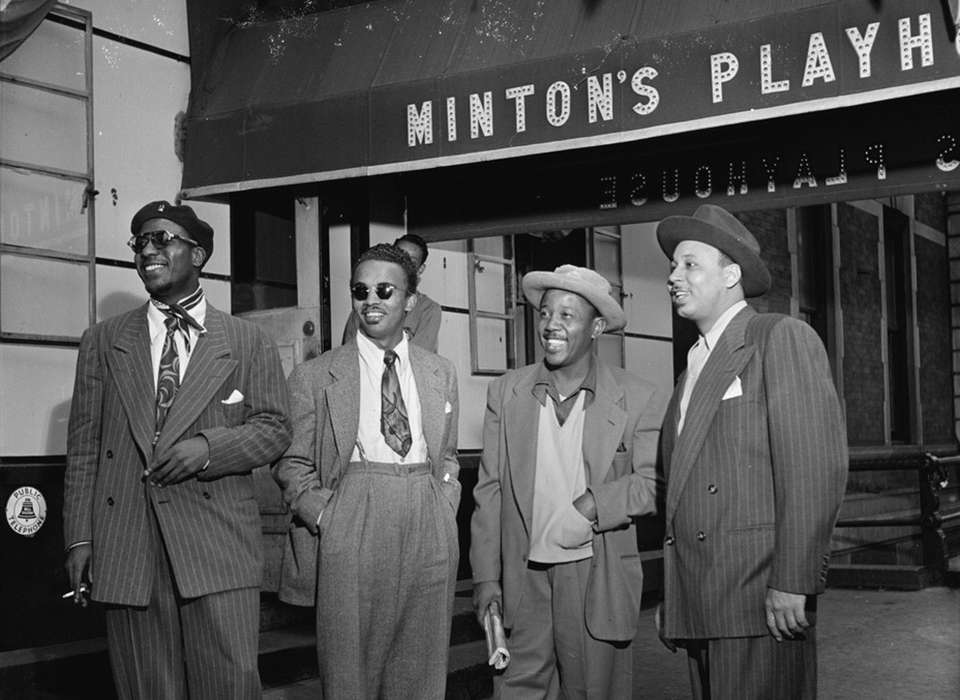This black-and-white photograph from possibly the 1950s features four African American men standing in front of Minton's Playhouse, a renowned music venue. The men are positioned beneath an overhanging awning that prominently displays the venue's name.

From left to right, the first man is wearing dark sunglasses and a black beret. He is dressed in a gray-striped, double-breasted suit with a patterned dark tie and a slight scarf around his neck. He holds a cigarette in his right hand. Next to him, the second man sports round dark glasses and a small mustache. He is smiling and is dressed in a light-colored suit with suspenders, paired with a white collared shirt and a short patterned tie. 

The third man, shorter than the first two, is in a loose-fitting light gray suit. He wears a white vest over a gray shirt and has a hand tucked into the pocket of his vest. He holds a rolled-up newspaper in his right hand. The fourth man, on the far right, dons a pin-striped, double-breasted suit. While it's difficult to discern his tie, it might be white or absent as he is slightly turned sideways. He is also wearing a cap.

Behind the men is the recognizable façade of Minton's Playhouse, distinguished by its white stone and brick architecture. The background includes additional intriguing details such as windows and stairs, indicative of the venue's bustling city environment. The overall composition and attire of the subjects suggest they could be musicians, captured in a moment of camaraderie outside this legendary establishment.